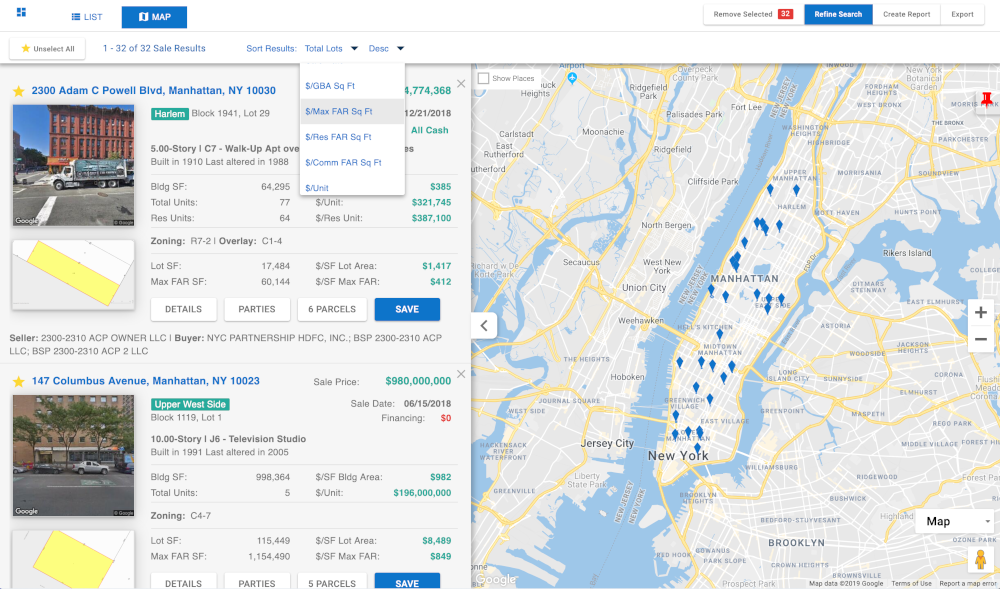This image showcases a real estate website interface focused on property listings in Manhattan, New York City. The screen is divided into two primary sections: the left side displays detailed property listings, while the right side features a map of Manhattan dotted with approximately 20 blue location pins.

On the left, the first listing presented is for the property at 2300 Adam C. Powell Boulevard, Manhattan, New York, 10030. The listing provides comprehensive details including seller and buyer information, pricing, zoning data, and a top-down map view highlighting the specific building within its urban block.

Below this, the second listing is for 147 Columbus Avenue, Manhattan, New York, 10023. Similar to the first, it offers extensive information on pricing, zoning, and an actual photograph of the location. Additionally, a top-down map view indicates the exact position of the lot.

The map on the right side of the screen shows the layout of Manhattan, with the highlighted pins corresponding to the various property listings available, facilitating an easy visual search for potential buyers.